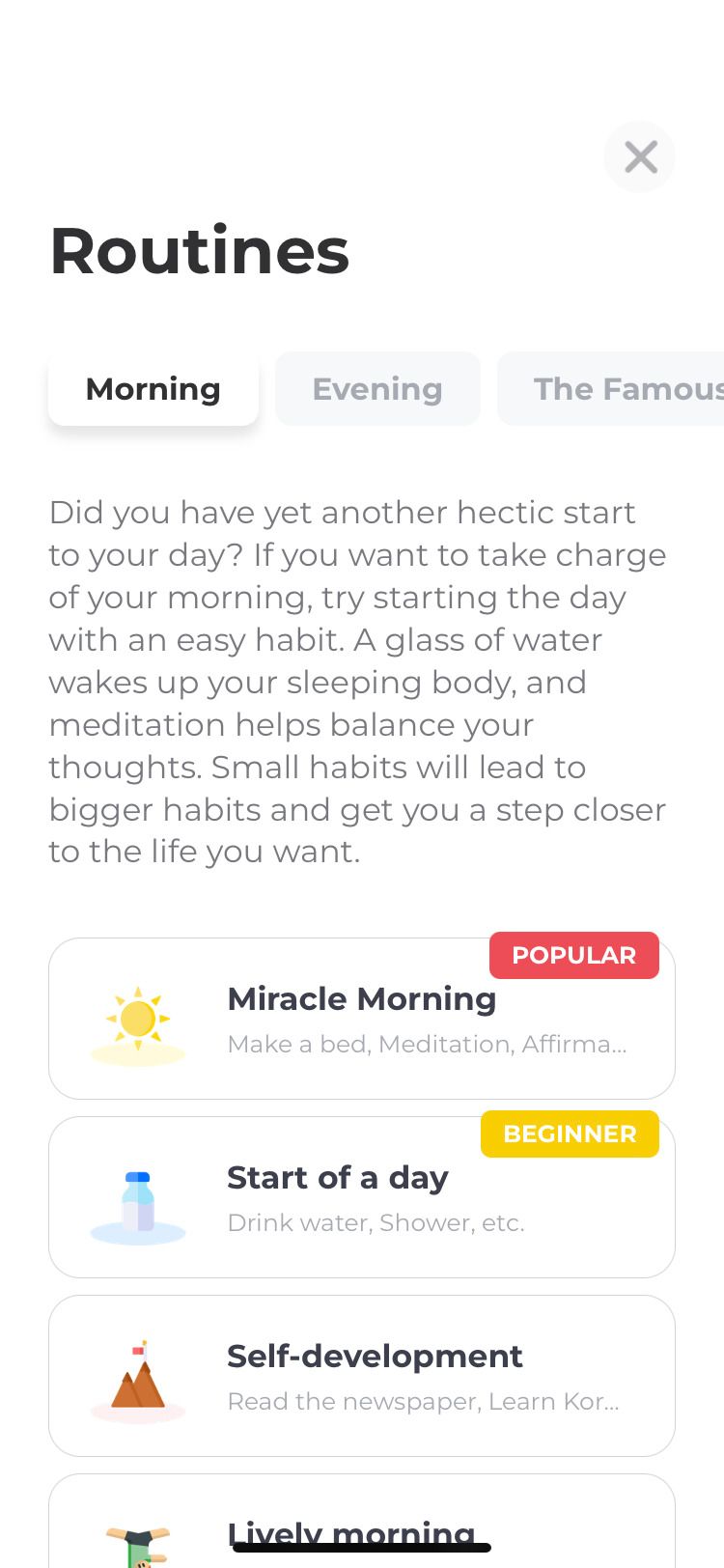The rectangular image is oriented vertically, with the longer sides extending from top to bottom. In the top right corner, there is an "X" enclosed within a faint circle. Prominently displayed in large black letters at the top is the word "Routines." Below this heading, there are three options listed: "Morning," "Evening," and "The Famous." Both "Evening" and "The Famous" are grayed out, while "Morning" appears to be selected.

A block of text follows, reading: "Did you have yet another hectic start to your day? If you want to take charge of your morning, try starting the day with an easy habit. A glass of water wakes up your sleeping body and meditation helps balance your thoughts. Small habits will lead to bigger habits and you get a step closer to the life you want."

Beneath this text, there are four boxes outlined with thin gray lines. The topmost box is labeled "Miracle Morning" and features a small sun icon on the left. It lists "Make a bed, Meditation, and Affirmation," and is marked as "Popular" in a red box with white text.

The second box is labeled "Start of a Day" with a water glass or bottle icon. It lists "Drink water, Shower, etc.," and is marked as "Beginner" in an orange box with white text.

The third box is labeled "Self-Development" and is illustrated with a mountain icon. 

The fourth and final box is labeled "Lively Morning" and depicts an individual exercising.